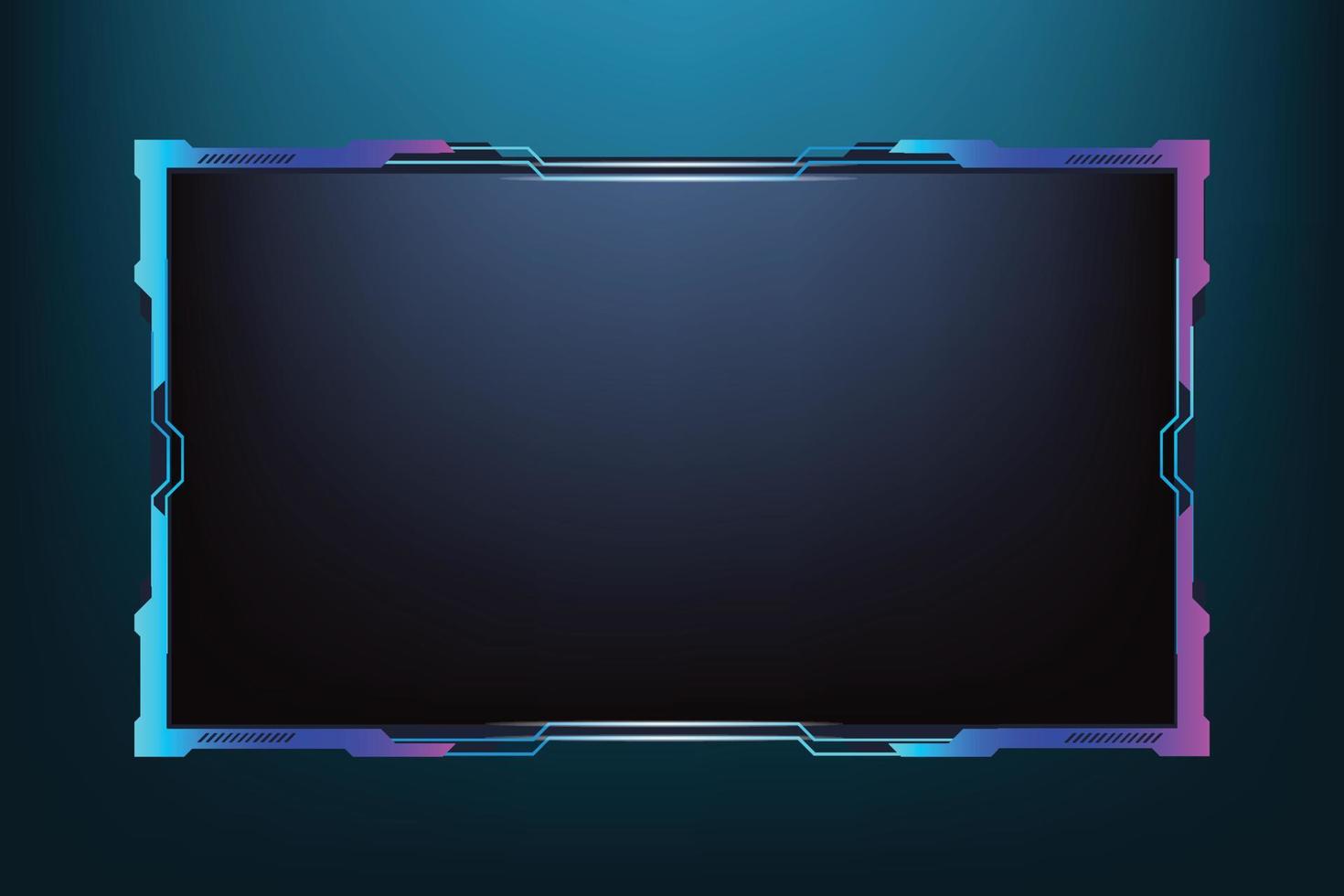The image features a futuristic, black flat screen TV with vibrant, cyberpunk-themed borders. The edges of the TV are adorned with a striking gradient that transitions from cyan to purple on the left, and purple to cyan and blue on the right. The upper and lower borders similarly blend light blue and pink hues. The sleek, sharp-edged design, reminiscent of Tron and created with precise, angular elements, enhances its high-tech appearance. These colored panels appear to float over an underlying black frame, adding depth and intricacy to the design. The TV itself is turned off, presenting a solid black screen. The background of the image is a dark blue-cyan gradient, with darker shades in the corners and sporadic cyan splotches, suggesting a digital, cybernetic ambiance. The design is completed with holes in the top and bottom borders, presumably for speakers, adding a functional layer to the aesthetic.